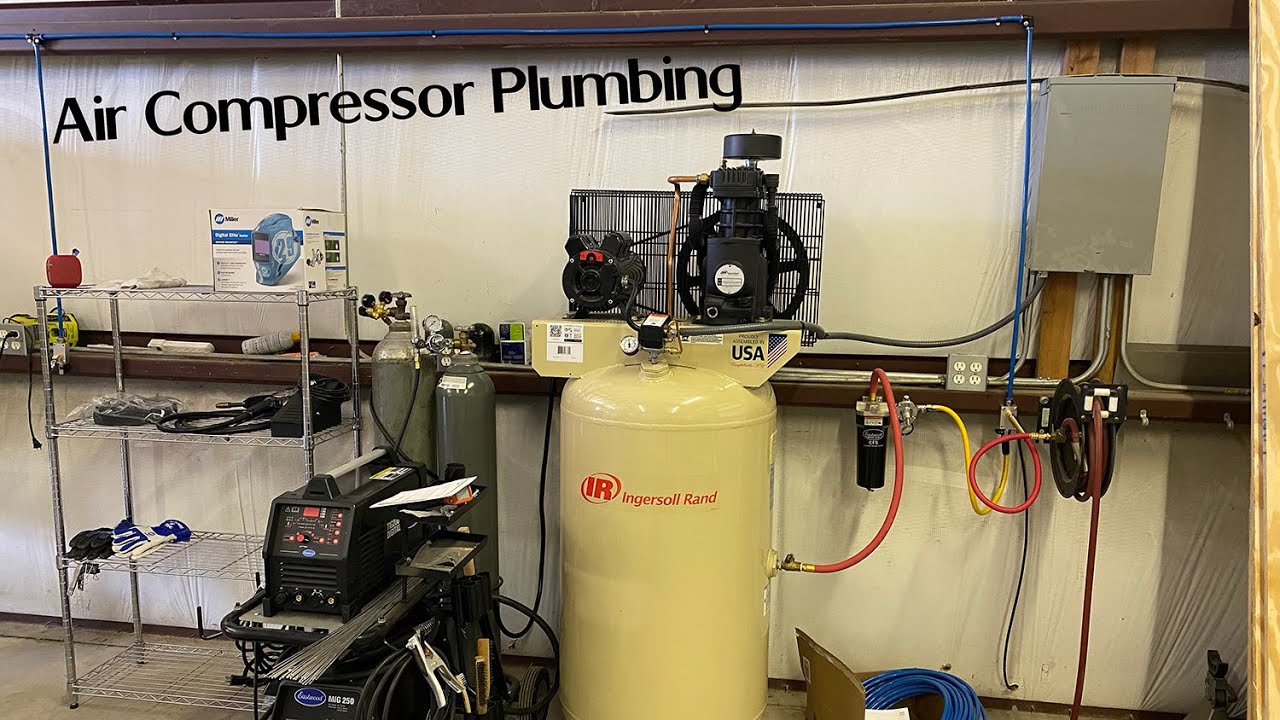The image, labeled "Air Compressor Plumbing," features a detailed setup of machinery against a wall in a machine room. Central to the image is a tall, yellow metallic cylinder akin to a propane gas tank, standing approximately four feet tall. The cylinder is marked with the red lettering "Ingersoll Rand," although the text appears somewhat unclear. Emerging from the right side of the cylinder is a red hose that connects to a unit mounted on the wall, presumably a control monitor or device.

Adjacent to this setup, the wall is dotted with various devices and components, likely associated with electrical pumps, all interconnected by an array of cords and tubing. To the left of the yellow cylinder, there are two oxygen tanks, positioned next to a computerized device, possibly a controller for the cylinders. Below this apparatus, a steel-gray shelf occupies the space, displaying an assortment of unidentifiable objects spread across its three visible shelves, including gloves and boxes.

The intricate network of hoses is further detailed: a red hose branches into a black box, which then transitions into a yellow hose before feeding into a silver box. From this silver box, a blue tube extends from the right side of the image, reaching up and across the top, towards the top left corner. The entire setup captures the elaborate and interconnected nature of the air compressor system within the machine room.